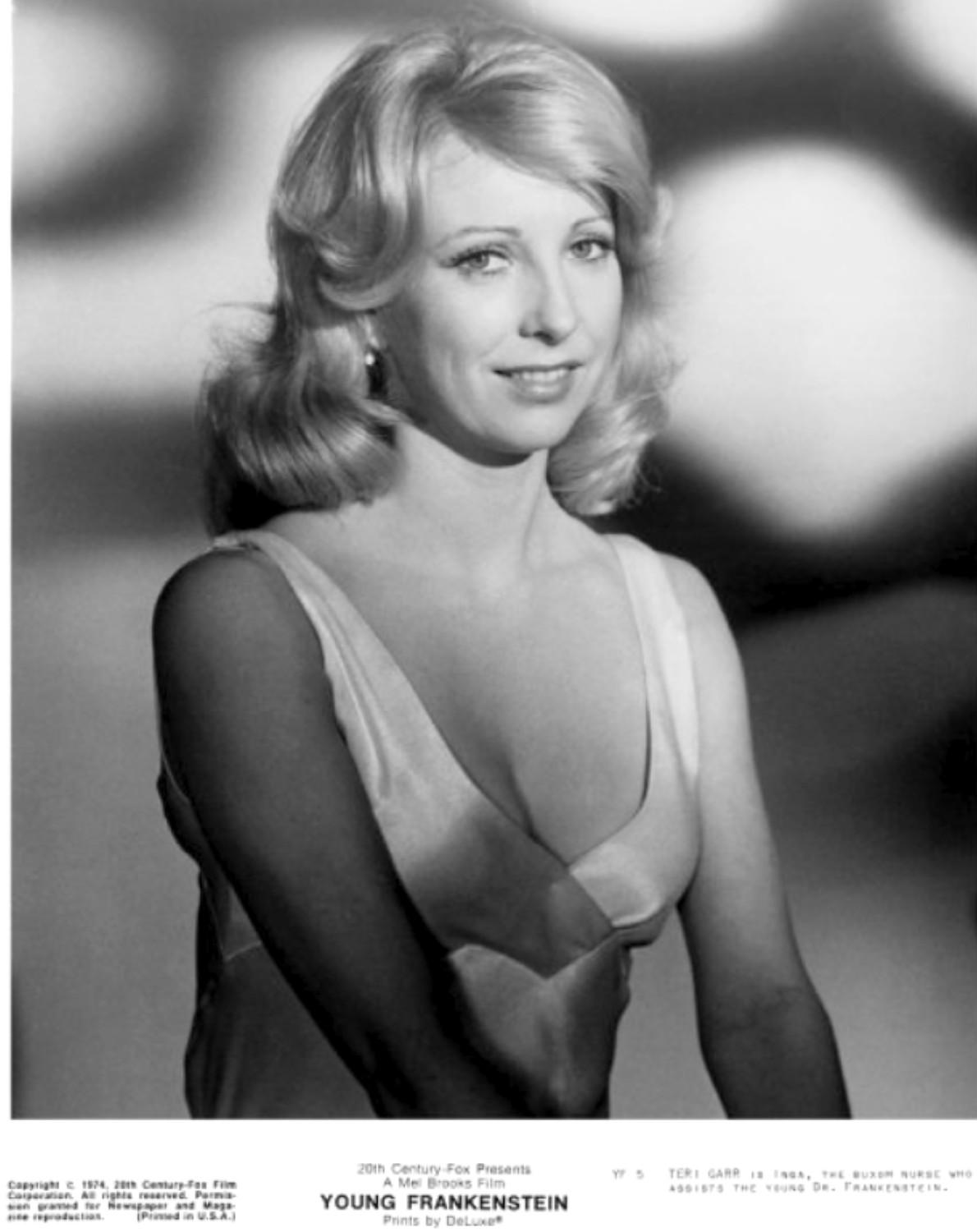This is a vertically aligned, black-and-white promotional photograph of a woman, likely an actress or model, taken from the waist up. She has shoulder-length, blonde hair that appears curly or wavy, reminiscent of a 1950s or 1960s style. She is dressed in a sleeveless, low-cut white or gray dress, possibly made of satin or silk, with straps that are thicker than spaghetti straps. Her arms are positioned in front of her, possibly resting on her lap, though her hands are not visible. The woman is smiling warmly at the camera, showing her teeth, with her body slightly turned but her face looking straight ahead. The background blurs into large blobs of white, black, and gray. Below the photograph is a series of text: in bold black letters, "YOUNG FRANKENSTEIN," and above it, "20th Century Fox presents a Mel Brooks film." Further details include "PRINTS BY DELUXE" in bold, with some finer, unreadable print flanking the main text. The bottom left corner reveals a small block of text that includes a copyright from 1974, while the bottom right mentions what could be the photographer's name and the name "Teri Garr" (consistent with the likely identity of the photographed woman).